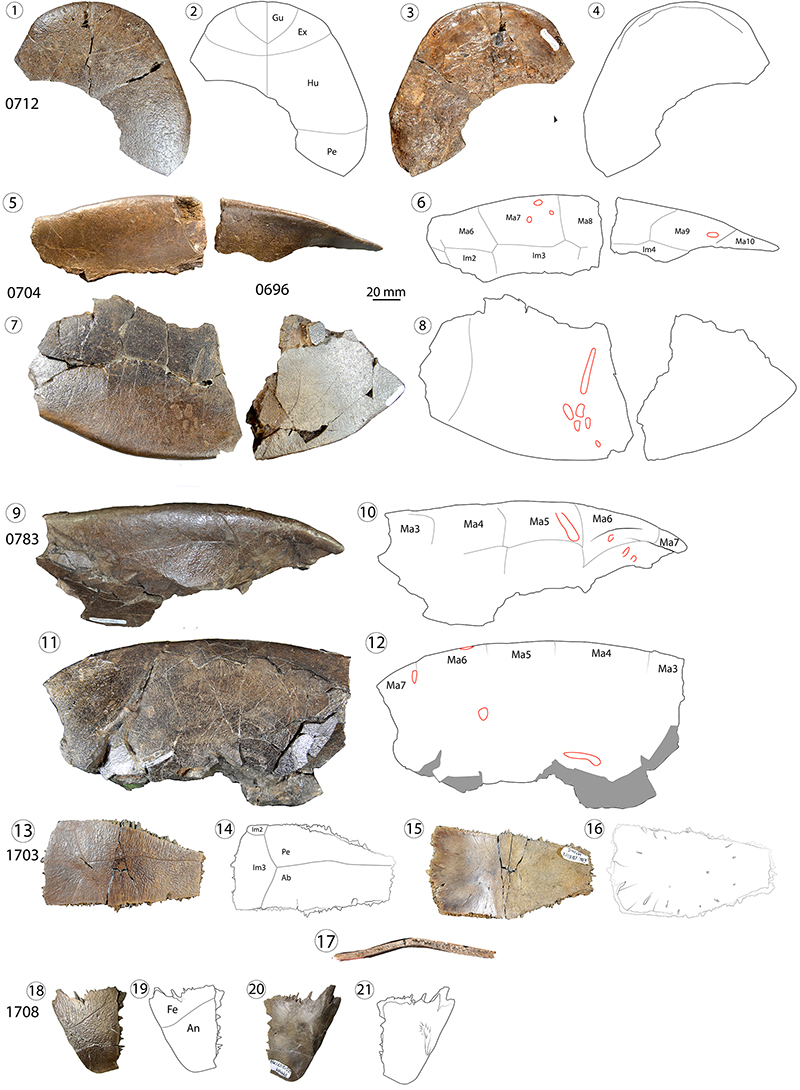The image depicts a detailed archaeological poster featuring 21 examples of fossils or bone fragments, each meticulously numbered from 1 to 21. Each example is presented in a combination of color and black-and-white photographs that show different aspects or orientations of the items. The poster starts with item number 1, labeled with the code 0712, showing a brown half-circle shape, potentially indicating a fragment or a partial fossil. 

Following that, item number 2 is a black-and-white image showing a similar orientation, while item number 3 is a brown version but facing in the opposite direction. Item number 4 is white, and item number 5 appears to be a broken tusk also in brown. Item number 6 mirrors it in black and white. Number 7 combines gray and brown elements, with number 8 in white directly to its right. This pattern continues with alternating brown and white representations for items 9 through 12 and beyond.

Each fossil or fragment includes a numerical designation and a correlating sketch on its right side, highlighting specific features with further numerical delineation. These annotations likely serve as reference points for cataloging and analysis, despite no text legible to casual observers. Visually, the items vary in shapes and sizes, ranging from half-moon shapes to potentially fractured stone-like implements. The detailed poster seems to break down each fossil into its components, using labels to map out cracks and other significant features, creating a comprehensive visual reference that aids in the study and comparison of these archaeological finds.